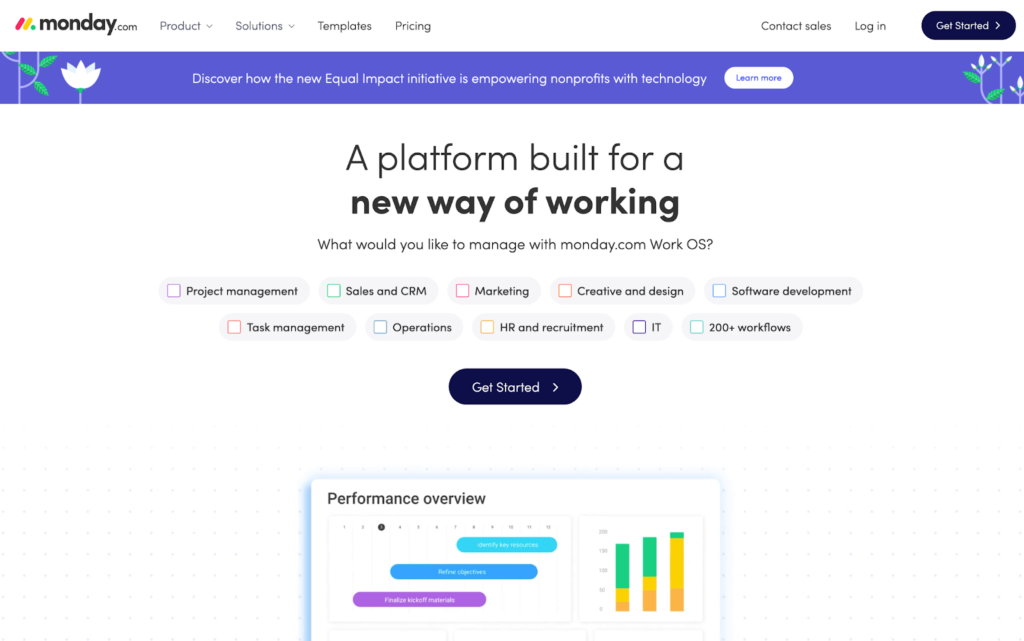The screenshot shows a webpage from monday.com. In the top-left corner, there are three elliptical, jellybean-shaped icons in red, yellow, and green, resembling traffic lights. Adjacent to these icons, "monday.com" is displayed in large, bold, black lowercase letters. To the right, there are four tabs labeled "Product" (with a drop-down arrow), "Solutions" (with a drop-down arrow), "Templates," and "Pricing."

Below this, a purple banner features a white tulip with green vines on its left side. The banner text, in white letters, reads: "Discover how the New Equal Impact Initiative is empowering nonprofits with technology." A white, elliptical button with purple letters saying "Learn More" accompanies this banner.

On the top-right corner of the page, there are additional tabs labeled "Contact Sales" and "Log In," along with a prominent "Get Started" button.

The central area of the screenshot has a white background with the following text in structured lines: "A platform built for a" (first line in black letters), "New Way of Working" (second line in bold black letters), and "What would you like to manage with monday.com work OS?" (third line in small black letters). Below this text, there are several categories with colored boxes for selection:

- Purple Box: Project Management
- Green Box: Sales and CRM
- Pink Box: Marketing
- Red-Orange Box: Creative and Design
- Blue Box: Software Development

On the second line of categories:
- Red Box: Task Management
- Blue Box: Operations
- Yellow Box: HR Recruitment
- Purple Box: IT
- Green Box: 200+ Workflow

Under these categories, a black button with white letters reading "Get Started" and a right-pointing white arrow is displayed. Finally, at the bottom of the screenshot, there is a chart labeled "Performance Overview."